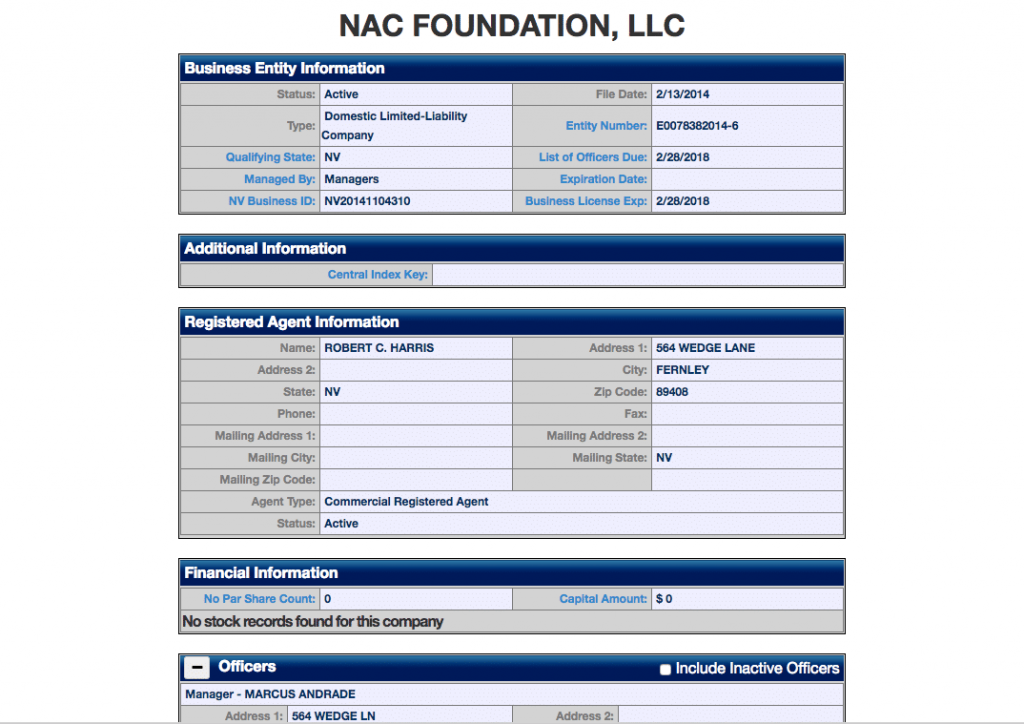The image is from a NAC Foundation LLC page, structured with multiple boxes categorizing various pieces of information. The first prominent box is labeled "Business Entity Information," detailing the following: 

- **Status:** Active
- **Type:** Domestic Limited Liability Company
- **Qualifying State:** Nevada
- **Managed by:** Managers
- **Nevada Business ID**
- **File Date:** February 13, 2014
- **Entity Number**
- **List of Officers Due**
- **Expiration Date**
- **Business License Expiration**

Another box titled "Additional Information" reveals:

- **Central Index Key:** Currently blank

Then there is the "Registered Agent Information" box, which includes:

- **Name:** Robert C. Harris
- **Location:** Nevada
- **Agent Type:** Commercial Registered Agent
- **Address:** Listed

In the "Financial Information" box, it is noted that:

- **Number of Par Share Count:** 0
- **Capital Amount:** $0
- **Additional Note:** No stock records found for this company

Additionally, there is a partially visible "Officers" box, which identifies:

- **Manager:** Marcus Andrade